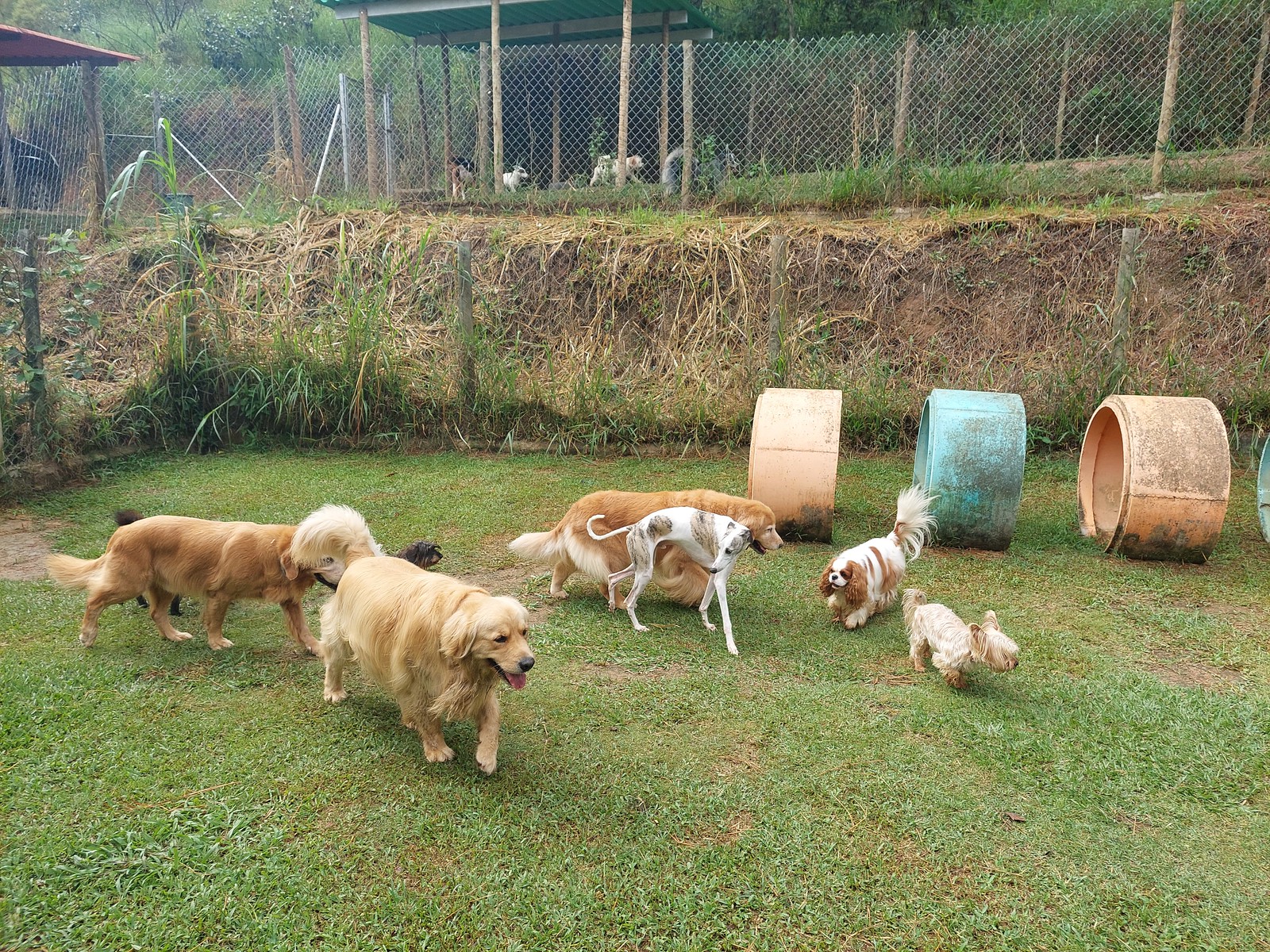The image depicts a group of seven dogs of various breeds including golden retrievers, a whippet, a Yorkshire terrier, and possibly a cocker spaniel, playing on a grassy field within a fenced-in yard. The central area where the dogs are playing features ceramic cylinders, possibly used as play tunnels, in shades of beige and turquoise. In the background, a hillside reveals another fenced enclosure containing more dogs. The fenced compounds, surrounded by a woodsy environment, suggest organized areas designed for the dogs, potentially dividing them into groups. Additionally, there is a structure in the background providing shade for the dogs, enhancing the setting's suitability as a dog compound.